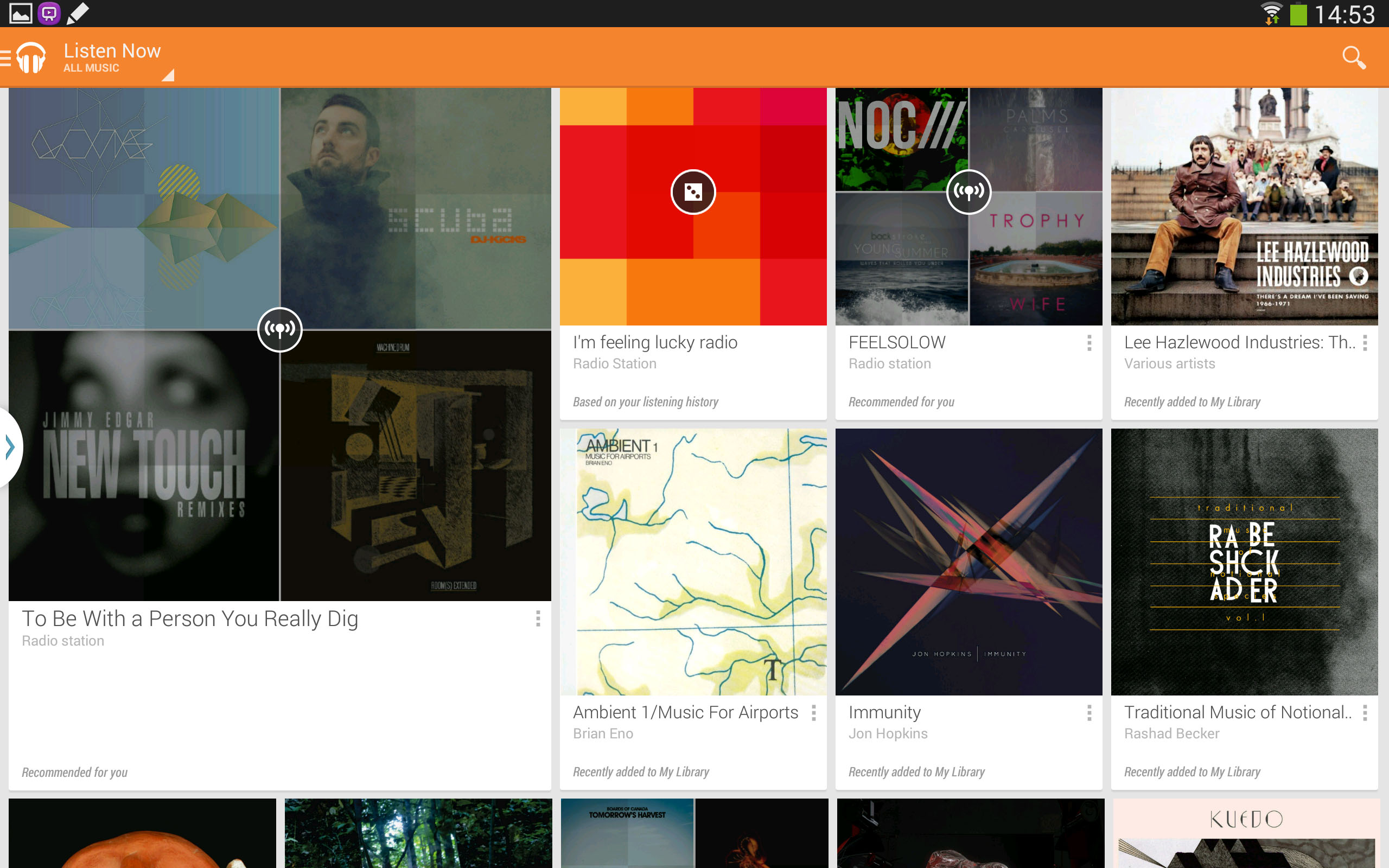The screenshot depicts a view from a tablet or computer screen. In the top right corner, the time is displayed in military format as 14:53, alongside a battery indicator showing a full charge. The main section features various clickable music album covers, including titles like "Phil's Sorrow," "Traditional Music," and "To Be With A Person You Really Dig." Multiple music selections are available for browsing. In the top left corner, there's a menu labeled "Listen Now All Music," suggesting it's a key navigation option. The site or application has a clean, white background, indicating it is a platform for exploring and listening to music.